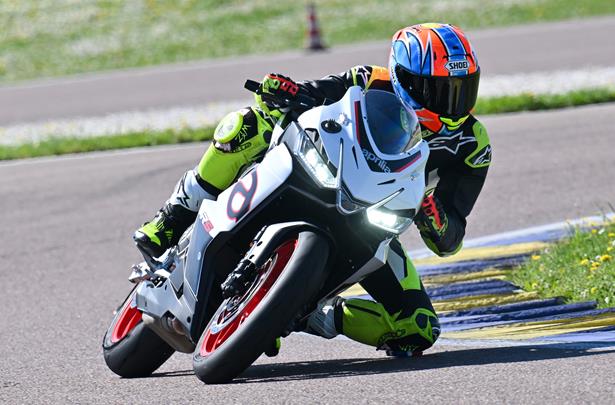This is a detailed photograph of a motorcyclist in mid-race, capturing the high-speed action and precision of the sport. The shot, taken from the front of the bike, reveals the rider angled sharply to the right, with the motorcycle precariously low to the ground, his knee brushing the pavement as he navigates a steep curve on the racetrack. The motorcycle, a striking combination of black and white with red rims and a white fender adorned with black accents, is at full tilt. The rider’s gear is vibrant and eye-catching: a helmet with blue, red, and white patterns, although the name inscribed on it is unreadable, and gloves in a bright lime green or yellow with red highlights. The uniform itself includes lime yellow pants, knee pads, and elbow pads, complemented by lime yellow boots accented with black and white. The outdoor setting of the racetrack features a paved track with grassy areas dotted with flowers and dandelions on the inside, and more grass on the outer edges, adding to the dynamic composition of the scene.